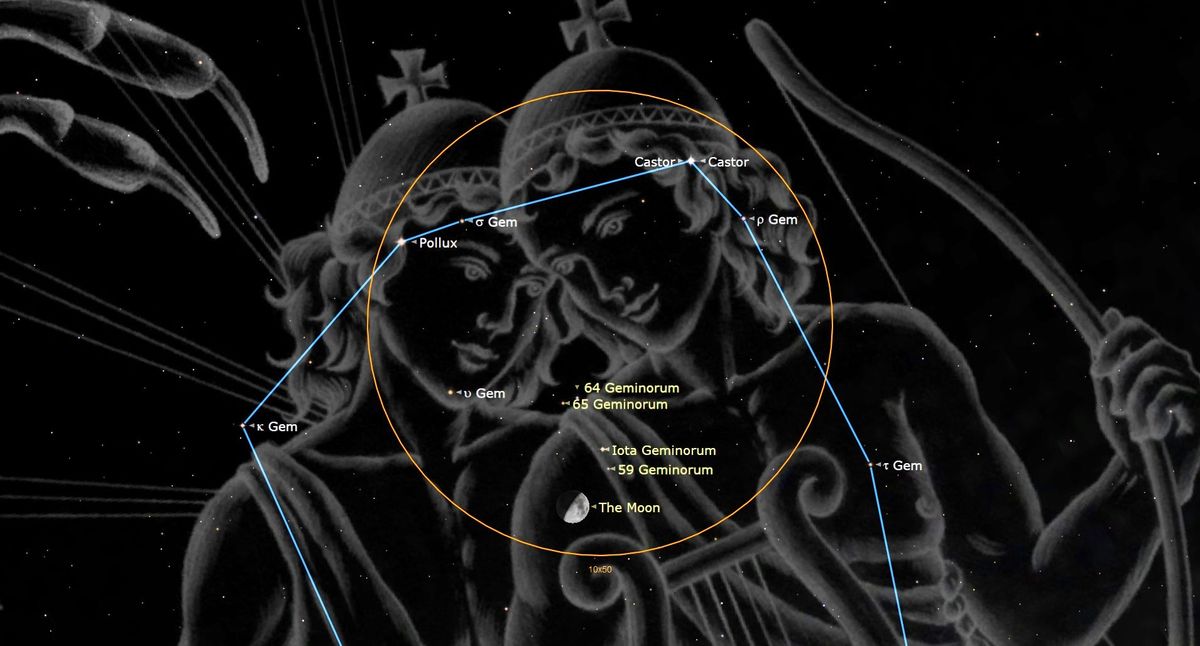In the image, there are intricate black and white depictions of the Gemini twins, represented as two youthful figures in a semi-classical style. One twin holds a bow, while the other carries a harp. They both wear distinctive caps adorned with crosses, suggesting possible mythological or Roman/Greek god references. Their attire is minimal, with exposed chests and arms, evoking images of togas. Surrounding them is a black background, contrasting sharply with their white relief.

Interspersed among the figures are geometric shapes and a star map, indicative of constellations. A labeled blue path meanders through the scene, pointing to celestial points such as K-Germ, Pollux, Alpha Gem, Castor, and other stars including 64 Geminorum, 65 Geminorum, Iota Geminorum, and 59 Geminorum. An orange circle encompasses these labels.

At the intersection where the twins' arms meet, there is another detailed feature: the moon. Additional elements include what appear to be tarantula-like insect legs with claws positioned in the top left corner. Altogether, the image blends classical mythology, astronomy, and abstract elements, creating a layered and detailed visual narrative.